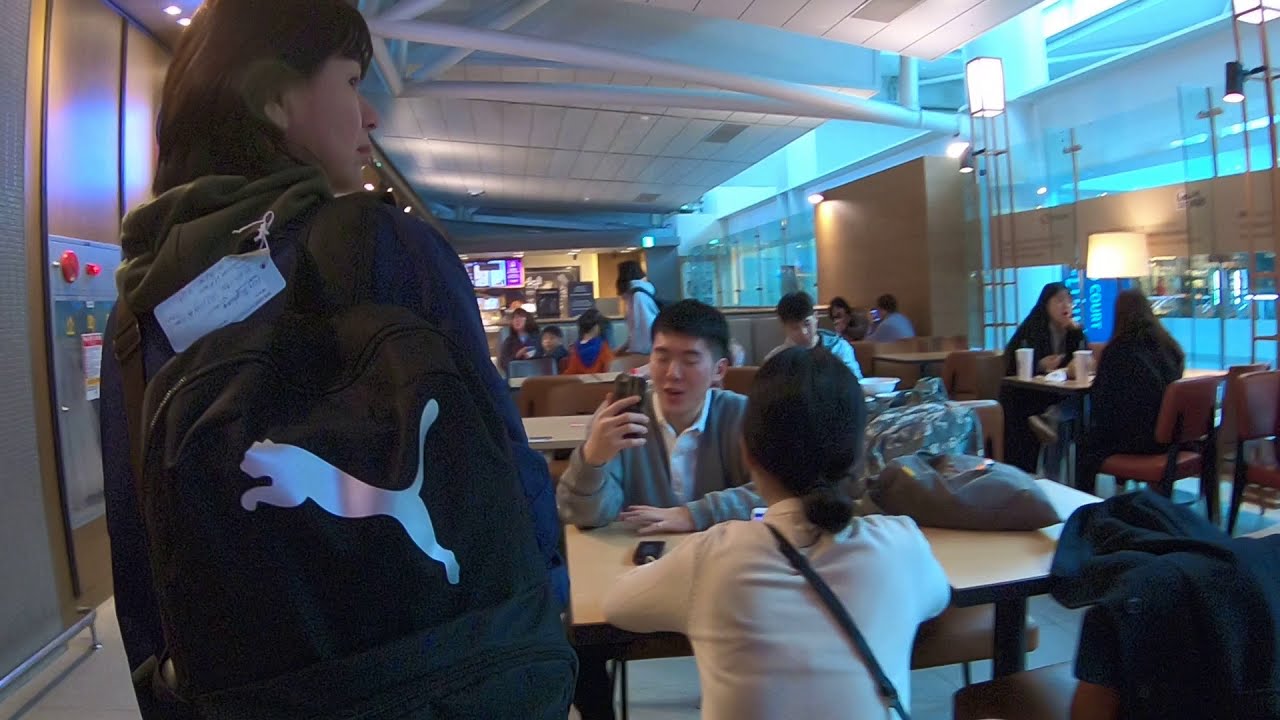The image captures a bustling food court or lounge area within a larger public building, possibly an airport or shopping mall. Dominating the foreground on the left side, a light-skinned Asian woman stands with her back to the viewer. She is distinguished by her black Puma backpack and black jacket. To her right, an Asian man in a gray jacket sits at a table, engrossed in his phone, directly facing the camera. Across from him, a woman with dark hair, wearing a white sweater and a bag, sits with her back to the viewer. More people of varying ethnicities, predominantly Asian, are visible throughout the space, seated at various tables, some engaged on their cell phones while others converse. 

The ambiance is bright with white layered ceilings featuring metal beams. Glass windows line the back, allowing natural light to filter in and offering a distant view of menu signs mounted on black chalkboard-like panels, suggesting various dining options. Wood paneling on the walls and a red emergency device lend a touch of structure to the scene. Further in the background, more patrons can be seen seated, their tables adorned with drinks. Overall, the image encapsulates the diverse and dynamic environment typical of a communal dining space.